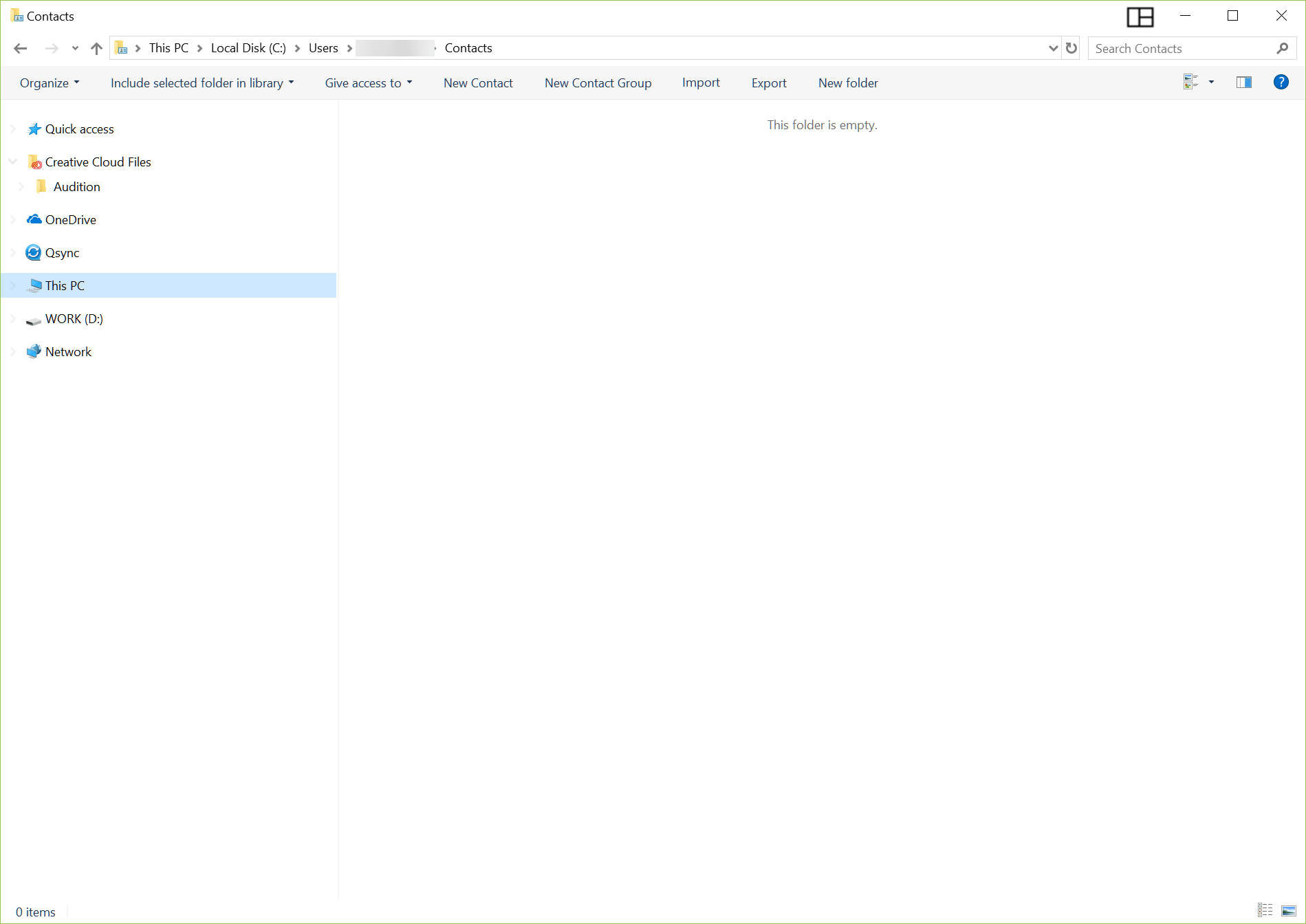This screenshot captures a view of a computer interface, specifically focused on the "Contacts" folder within a file explorer window. The interface is framed by standard window control buttons in the top right corner, including options to minimize, maximize, or close the window.

At the top left corner, the word "Contacts" designates the active folder. Directly beneath this title, navigation tools are available, including left and right navigation buttons and an up arrow for directory traversal. Adjacent to these buttons, a small folder icon leads into a breadcrumb path displaying "This PC > Local Disk > Users," with the username obscured by a rectangular blur. The path culminates in the "Contacts" directory, reaffirming the current location within the interface.

To the far right, below the window control buttons, a search bar labeled "Search Contacts" presents a search functionality dedicated to the contents of the "Contacts" folder.

Beneath these navigation tools, a horizontal, grayed-out toolbar spans the width of the interface, containing multiple tabs organized from left to right. These tabs include "Organize," "Include Selected Folder in Library," "Give Access to," "New Contact," "New Contact Group," "Import," "Export," and "New Folder," offering a variety of management and organizational options for the user.

Along the left side of the window, a vertical menu presents additional navigation entries, such as "Quick Access," "Creative," "Cloud Files," "Audition," "OneDrive," "QSync," "This PC," "Work," and "Network." "This PC" is currently highlighted, indicating its active status within the menu.

The main content area, situated toward the center and extending to the right side of the interface, displays a message: "This Folder is Empty," suggesting that there are no contacts currently saved in this location. The rest of the background remains white and unoccupied, maintaining a clean and uncluttered appearance.